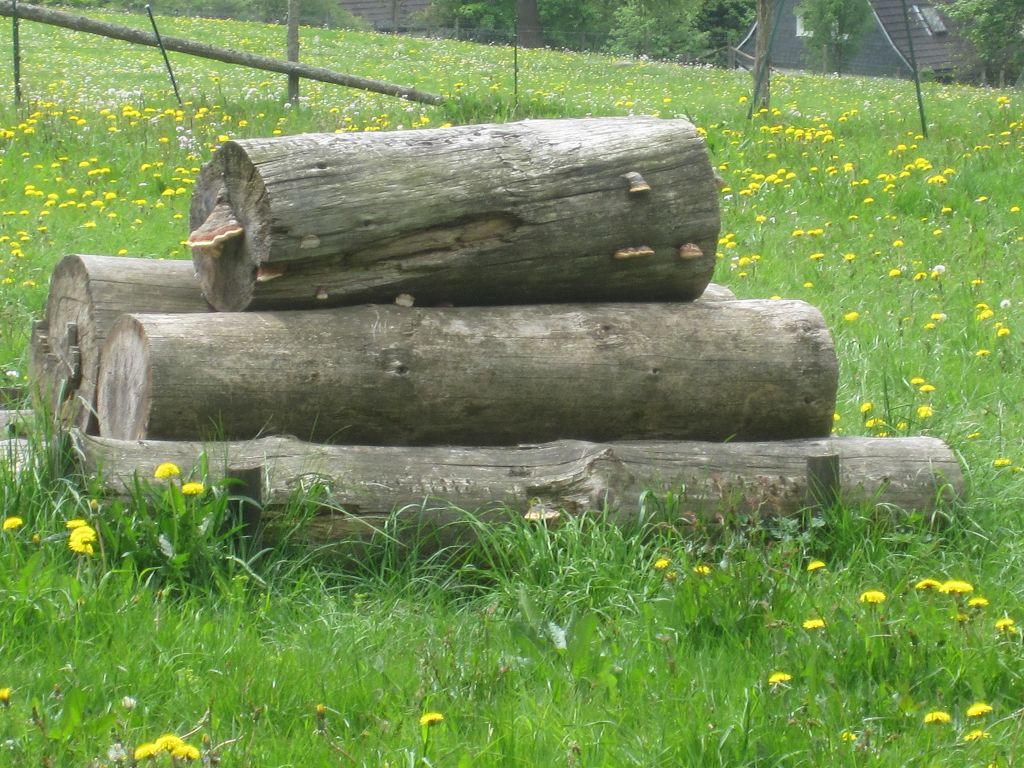In this photograph, we see a serene rural scene with a stack of large, dark gray logs lying in a lush, green grassy field. The logs, which vary in both length and thickness, are arranged in a pyramid, with the thickest one at the bottom and progressively smaller ones stacked on top. The logs appear heavy and rugged, hinting at their natural origin. The field is dotted with numerous yellow dandelions and some white flowers, adding a vibrant touch to the greenery. The grass itself is tall and verdant, contributing to the bucolic charm of the scene.

In the background, halfway up the rising hill which slopes towards the camera, there is an old gray house with white trim and windows, partially obscured by surrounding trees and bushes. The house sits quietly amongst the greenery, enhancing the secluded atmosphere of the location. Behind the logs, a barbed wire fence stretches across the field, marking a boundary and adding a rustic element to the landscape. The overall composition captures a peaceful, rural setting with a mix of natural elements and a hint of human habitation.